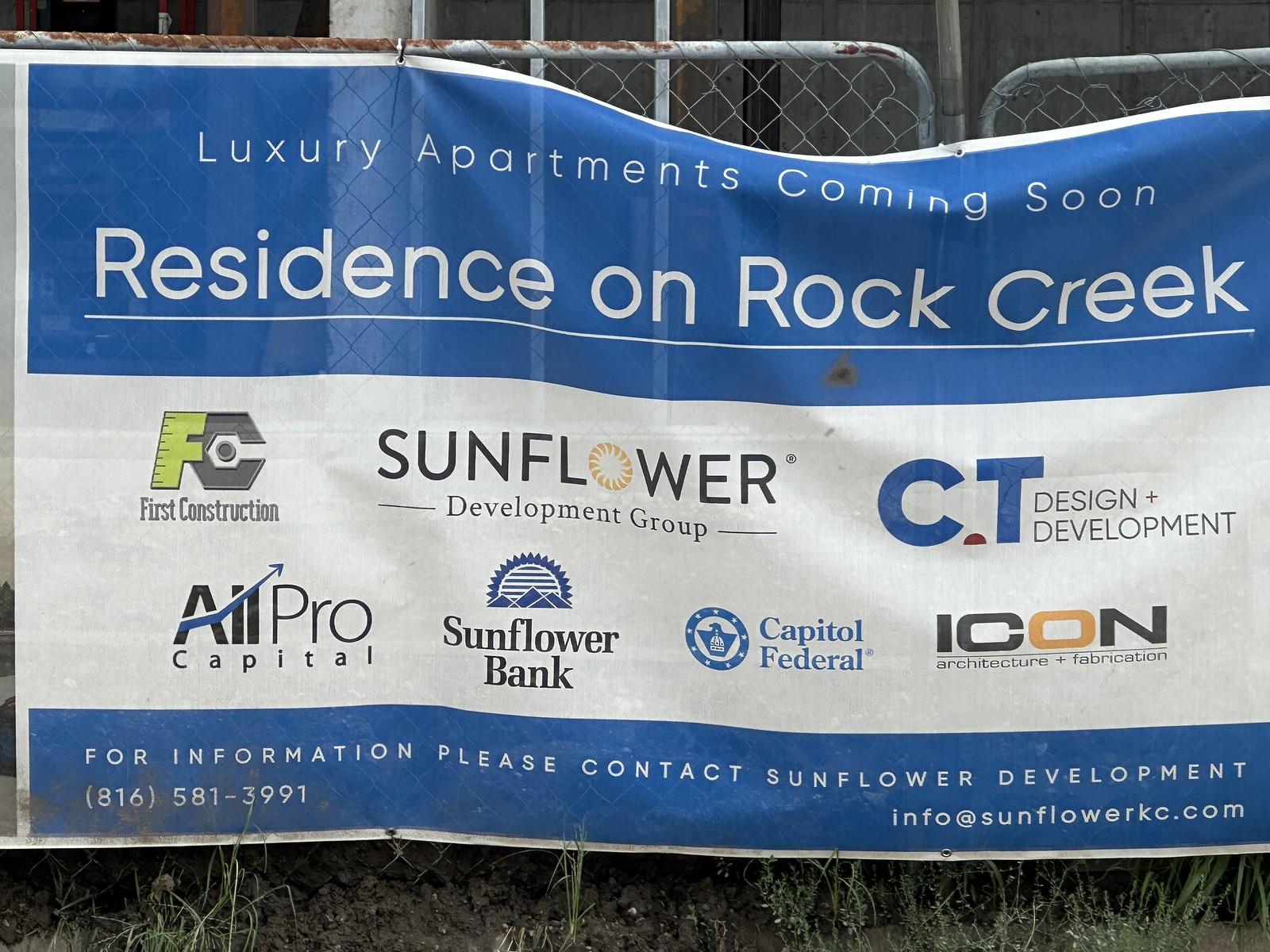This image depicts a disheveled banner hung on a rusty chain-link fence, situated in the foreground of an apartment complex. The banner, partially detached on the upper right side and slightly sagging, features a prominent blue rectangular block with white text announcing, "Luxury Apartments Coming Soon, Residents on Rock Creek." Below this, various company logos are displayed, indicating the entities involved in the development: First Construction (FC), Sunflower Development Group, CT Design Development, All Pro Capital, Sunflower Bank, Capital Federal, and Icon Architectural Fabrication. Each logo is distinct, with colors of blue, yellow, green, and black against a white background. At the bottom of the banner, another blue strip contains the contact information for Sunflower Development, including a phone number, 816-581-3991, and an email address, info@sunflowerkc.com. The area beneath the fence shows patches of dirt and weeds, contributing to the overall unkempt appearance of the scene.